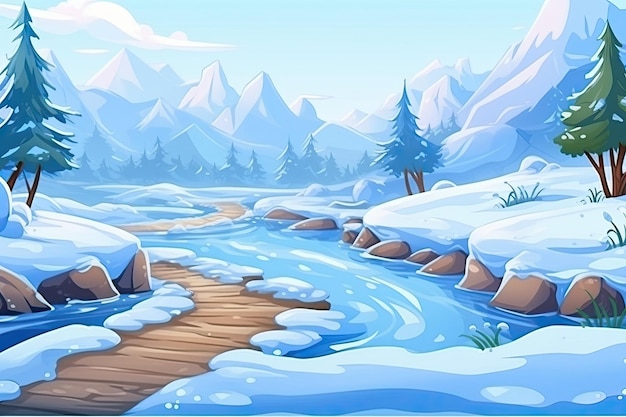This digital artwork depicts a serene snowy mountain region under a clear, light blue sky with a single fluffy cloud. Prominently featured is a gently curving dirt path resembling wood, possibly a bridge, that winds alongside a flowing river. The river, lined with rocks and brown riverbanks, gracefully traverses the scene from the foreground to the distant background where it appears to merge or go under the snow. Pine trees are scattered throughout, with several close to the viewer on both the left and right sides, forming lines that stretch into the distance. Beyond these trees, a grey mountain range rises, capped with snow, completing the tranquil landscape.